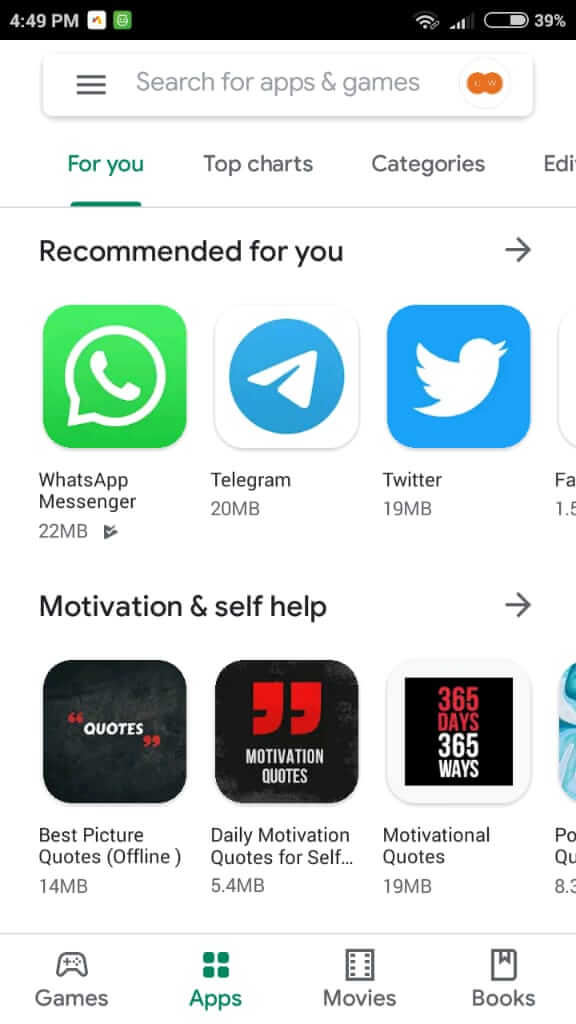This image shows a mobile phone screen displaying a web page, likely an app store. At the top of the screen, standard phone indicators such as battery level, signal strength, carrier signal, Wi-Fi status, and the current time are visible. Below these indicators is a search bar for finding apps and games, accompanied by a menu icon represented by three horizontal lines on the left side and two overlapping red dots resembling the MasterCard logo on the right side.

Directly underneath the search bar, the interface includes navigational tabs with 'For You' currently selected, followed by 'Top Charts,' 'Categories,' and a partially visible tab labeled 'EDI...,' which seems to be cut off, possibly indicating 'Edit.'

The main content beneath these tabs is titled "Recommended for You," showcasing various app suggestions including WhatsApp, Telegram, and Twitter. Further down, there is a section dedicated to 'Motivation and Self-Help' options featuring apps or resources related to quotes and motivational content.

At the bottom of the screen, there are four icons representing different sections of the store: Games, Apps (which is highlighted), Movies, and Books. The structure and content suggest an interface designed to help users discover and download various apps, entertainment, and self-help resources.